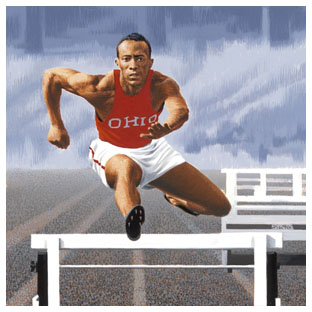This image, which appears to be a painting, captures a dynamic moment of a black male athlete, possibly Jesse Owens, mid-jump over a white hurdle on a racetrack. The runner is centrally positioned and facing the camera. He is clad in a red sleeveless tank top emblazoned with "Ohio" in white letters and sports white shorts featuring a thin red stripe down the sides. His footwear consists of black running spikes. The athlete’s right foot is forward with the sole visible, while his left leg trails behind him. His left hand is extended forward, and his right arm is bent at the elbow, positioned behind him. He has very short black hair. 

The hurdle he leaps over is white with black markings on the sides. The backdrop includes a gray racetrack with visible white lines, stretching beneath and behind him. The upper portion of the image suggests the presence of a stadium or stands, though these are portrayed with a blurred, indistinct appearance. On the right side of the painting’s background, there might be a white wooden bench, and the scene is set against a cloudy gray sky. The painting is square-shaped, presenting a detailed and vibrant depiction of athletic prowess and historical significance.